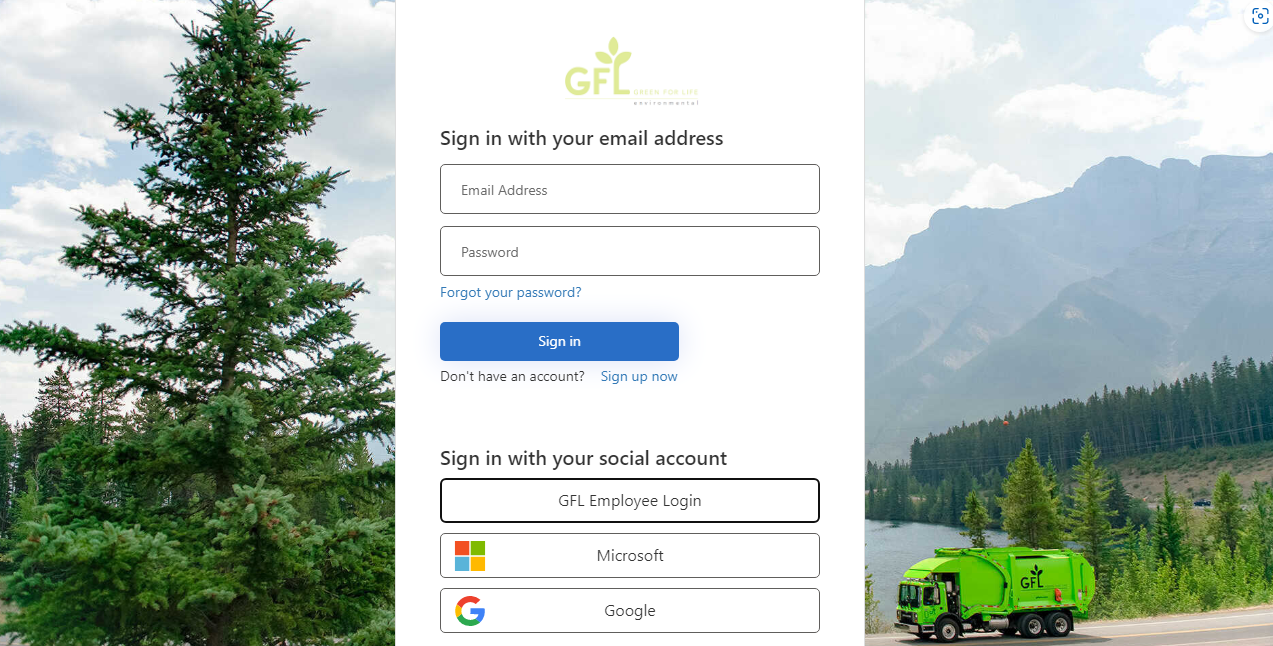The image depicts a login screen for a platform, with the acronym "GFL" prominently displayed at the top against a white background. To the right of "GFL," there is additional text in a pale green font, which is difficult to read due to the font color. Below the header, there is a prompt for users to "Sign in with your email address." 

The login form consists of two input fields: the first field, labeled "Email Address," and the second field, labeled "Password." Beneath these fields is a link in blue text that reads "Forgot your password," followed by a dark blue button labeled "Sign In."

Further down, the screen prompts users who do not have an account with the message, "Don't have an account?" and provides a "Sign Up Now" link in blue text to the right. 

At the bottom of the screen, there is a section titled "Sign in with your social account." It includes options for alternative login methods: the first button for "GFL Employee Login," followed by buttons for "Microsoft" and "Google," each accompanied by their respective company logos on the left.